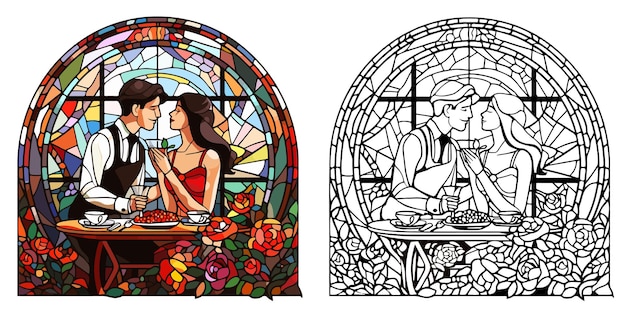The image depicts two nearly identical illustrations set against a stark white background. Both illustrations feature a man and a woman dining together in a romantic setting, captured in a stained glass window motif. On the left, the scene bursts with color; intricate designs of greens, browns, reds, pinks, and yellows dominate, woven into an almost lifelike stained glass window with vibrant roses and other flowers at the bottom. The couple, illustrated in a cartoon style, sit close together at a wooden table, nearly nose-to-nose as if about to kiss. 

The woman, with long flowing brunette hair, is dressed in a red dress with straps, holding a wine glass. The man, with wavy brown hair, is wearing a white button-down shirt paired with a black vest, tie, and an apron, giving him the appearance of a waiter. A red dish, white teacups on coasters, and glasses of wine add to the detailed dining scene. 

On the right, the exact same image is presented but stripped of its vibrant colors, rendered entirely in grayscale. This black and white illustration mirrors every detail of the colorful version: the couple’s attire, their intimate posture, the elaborate floral designs, and the dining elements, providing a clear contrast between the vividness of color and the simplicity of monochrome.